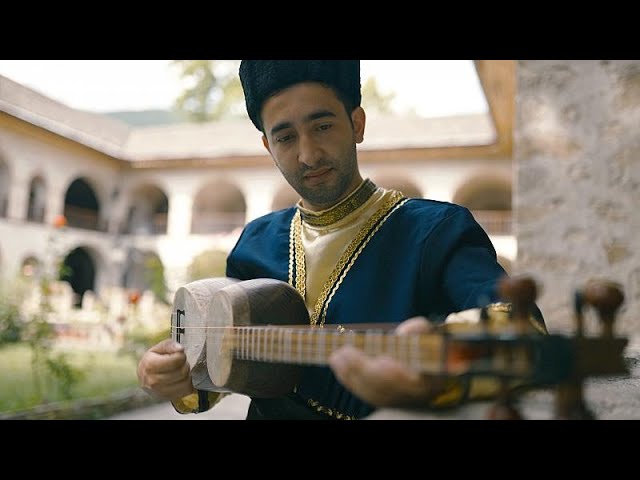In the center of the photograph, there is a mid-aged man with olive-toned skin, playing a unique musical instrument that resembles a guitar fused with two round drum-like components, possibly bongos, attached to the strings. He is wearing an ornate, dark blue, long-sleeve, silk suit adorned with gold accents, over a gold shirt, which hints at traditional Indian attire. The man also sports a tall, black, circular hat made of thick wool or fur-like material, reminiscent of Russian styles. The man faces the camera, and his stance brings the focus onto his detailed outfit and the unusual instrument. His beard looks freshly shaven with slight regrowth. The background, though blurred, reveals a two-story clay building with architectural elements reminiscent of the Colosseum, along with some indistinct greenery and trees, enhancing the scene's exotic ambiance. There is no text in the image.